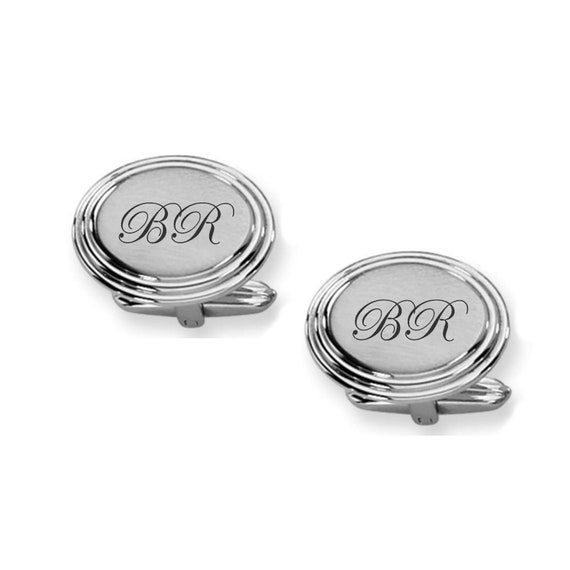This image features a pair of matching silver cufflinks set against a plain white background. The cufflinks are oval in shape, and due to the image being black and white, the silver appears in various shades of gray. Each cufflink consists of a smooth, solid silver center bordered by two raised, grooved ridges. In the middle of the solid silver area, there is an elegant monogram of the initials "B" and "R" in an almost black shade, crafted in a fancy, cursive script. The cufflink toggles are visible beneath each piece. These cufflinks appear to be designed for formal wear, adding a personalized touch with the engraved initials, likely suggesting they are a gift for someone with those initials.